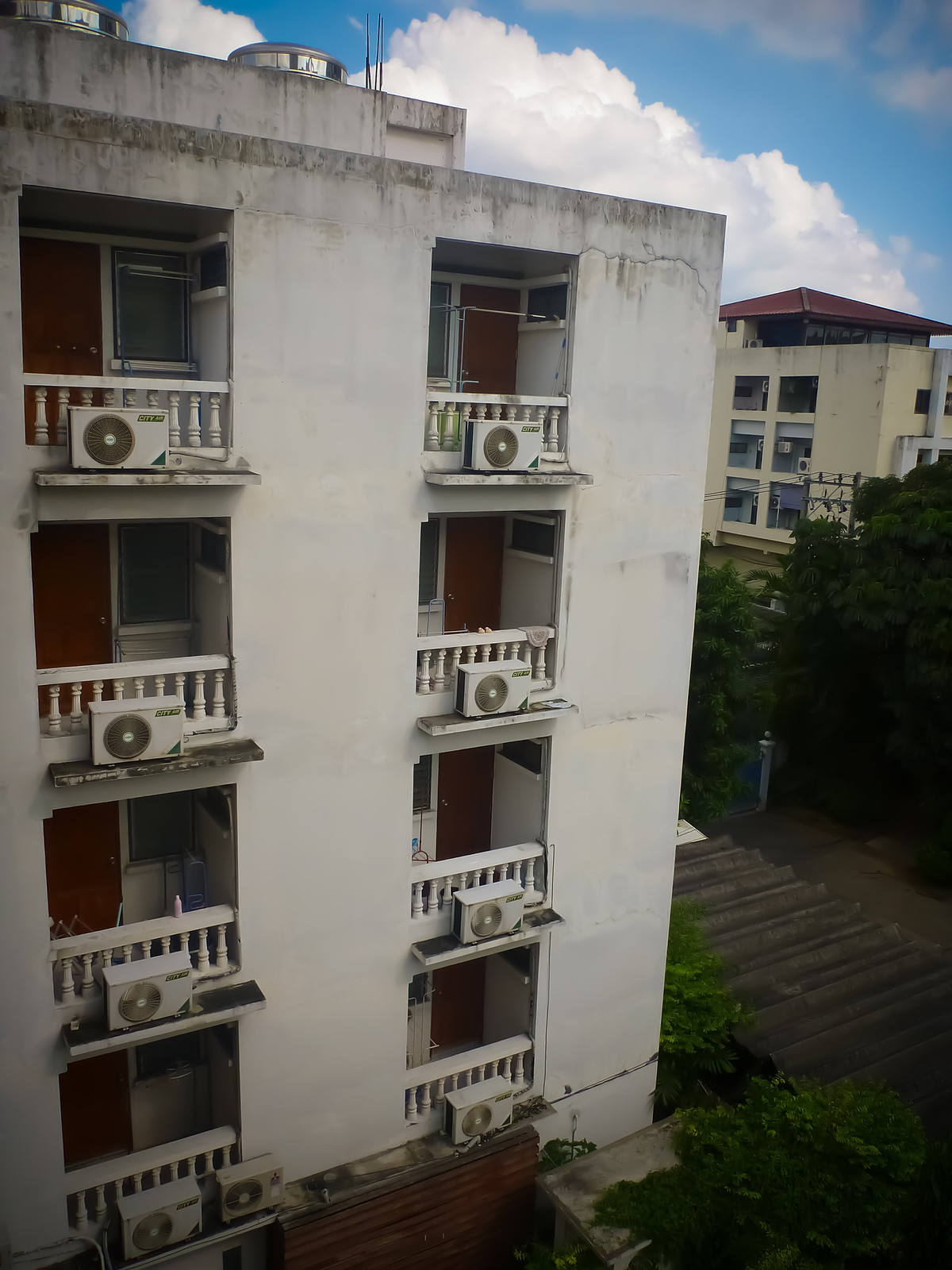This photo features a weathered, five-story tall apartment complex made predominantly of white concrete that has become quite dirty and deteriorated, especially towards the top. The building's facade is lined with two vertical columns of four balconies each, making a total of eight balconies. Each balcony is equipped with identical wooden guardrails featuring ornate, chess piece-like Italian-style pillars. They all have the same rectangular air conditioning units that are mostly white with a green triangle on the bottom right-hand corner, labelled "GTOF3." Doors accompanying these balconies are uniformly red, with green blinds decorating the windows. A closed, rusted garage door is visible at street level. The scene includes a manila-colored building in the far right background, and contrasted against the vibrant blue sky with fluffy clouds are full-canopied trees and shrubs surrounding the structure, adding a touch of greenery to the urban setting.